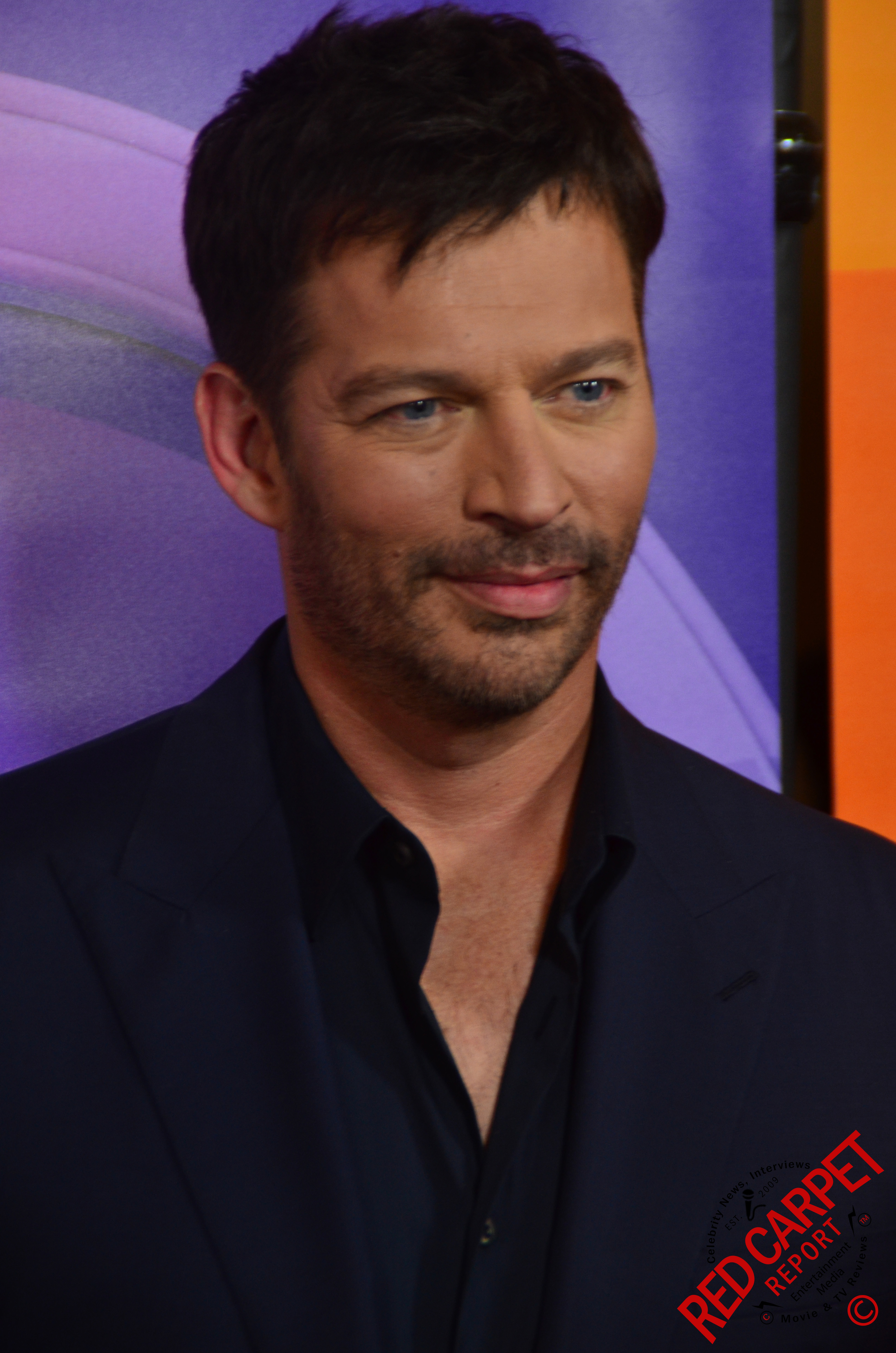The image features a portrait of a happy-looking man, smiling subtly with a lopsided, closed-mouth smile. He has prominent deep blue eyes and a well-groomed stubbly beard and mustache. His hair, either black or very dark brown, is styled in a medium length and slightly messy, combed to the side. The man appears to be in his 30s and is wearing a navy blue button-down shirt, slightly unbuttoned at the top, underneath a matching navy blazer. The photo captures him from the chest up as he gazes slightly to the right. 

The background is a mix of purple and orange hues, featuring a framed poster with purple and lighter purple elements, including a curved stripe across it. An orange strip runs along the right side of the image, stretching from the top to the man’s shoulder. In the bottom right corner of the image, the words "Red Carpet Report" are written diagonally in red text, accompanied by a copyright symbol. This visually cohesive background highlights the subject, accentuating his pleasant demeanor and confident presence.